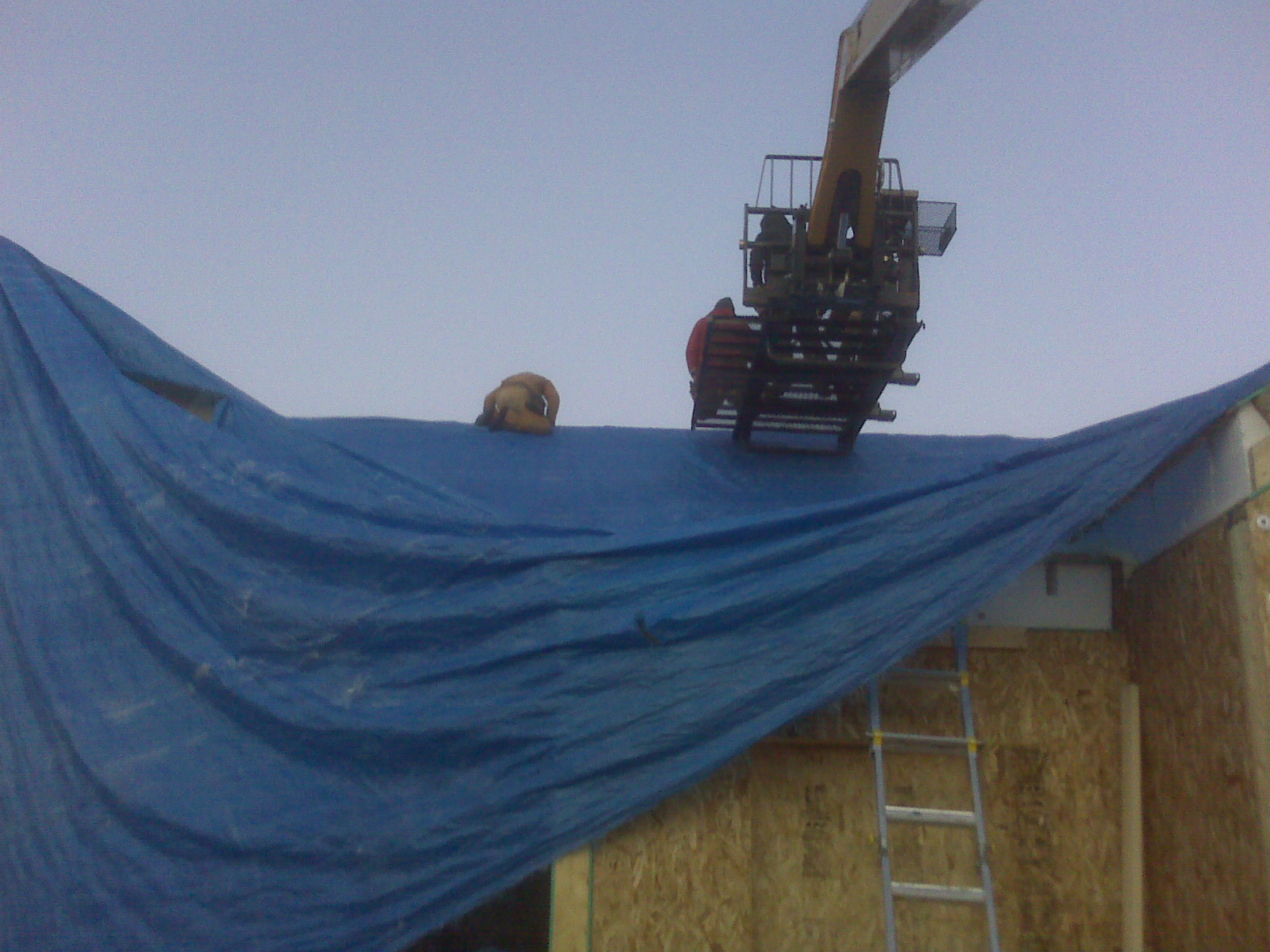The image depicts an active construction site under a clear blue sky. Dominating the upper right portion, a yellow crane arm supports a black metallic platform where two workers stand—one wearing red, the other in black. A third worker, dressed in yellow, is kneeling on the unfinished structure to the left. The construction area at the bottom right features visible plywood walls and a leaning silver extension ladder. A large blue tarp, draped diagonally from the left side of the image toward the bottom right, partially conceals the structure beneath, exposing sections of wooden framing and white trim. The scene is filled with various colors, including numerous shades of blue, gray, silver, brown, black, and red, contributing to the detailed and vibrant depiction of the construction environment.